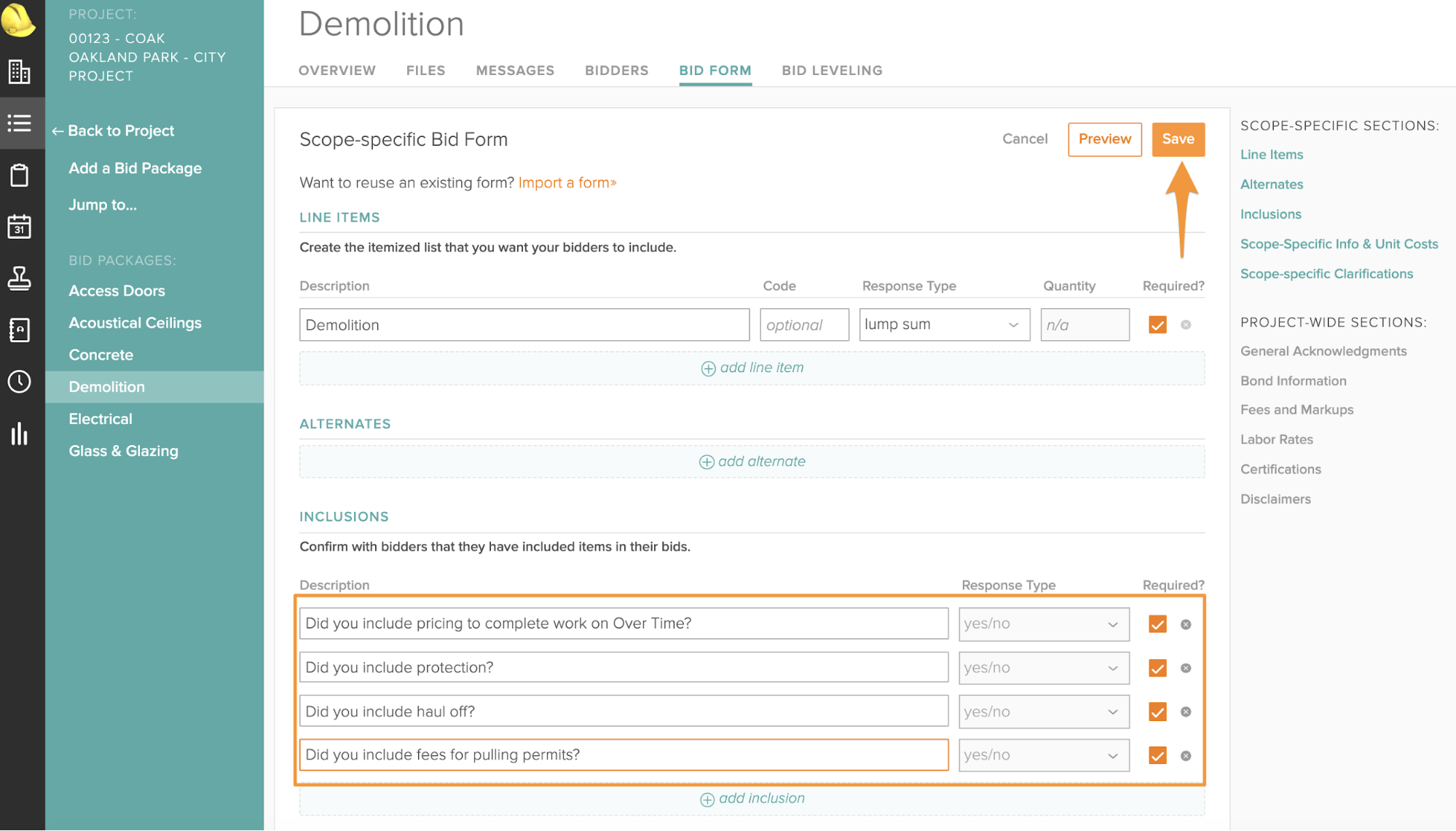The image features a detailed view of a construction project management interface. 

On the left side, against a white background, there is a vertical array of construction-related icons: a white construction helmet, a yellow construction helmet, a building, three dots with three lines alongside it, a clipboard, a calendar date, a stamp, a notebook, a clock, and a bar graph.

To the right of these icons, the background transitions to a bluish hue. At the top of this section is gray text that reads "Project," followed by white text that says "00123." Below this, it details a specific project named "Oakland Park City Project." Further down, there is an option to "Add a Bid Package" and a transition back to a gray-colored section titled "Bid Packages." Listed under this are various construction categories: "White Access Doors," "Acoustic Ceilings," "Concrete," "Demolition," "Electric/Electrical," and "Glass and Glazing."

On the far right side, the background color changes to black. At the top, "Demolition" is prominently displayed in white text. Below this, gray text labels different sections: "Overview," "Files," "Messages," "Bidders," "Bid Form" (underlined in blue), and "Bid Leveling." There are also options for "Scope Bid," "Scope Specific Bid Form," and choices to "Use an Existing Form" or "Import a File." At the bottom right, there are "Cancel," "Preview," and "Save" buttons, with the "Save" button highlighted in orange and indicated by a downward arrow.

In the lower section, the description area focuses on "Demolition," detailing options for a lump sum and various inclusions. There are fields for alternative bids, inclusions that need confirmation with bids, and a highlighted section in orange at the bottom. This section contains questions regarding whether pricing for overtime work, protection, haul-off, fees, and pulling permits are included, with required checkmarks in orange indicating these fields must be completed.